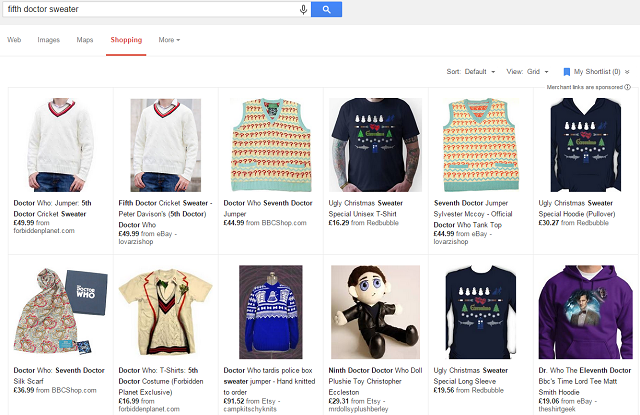In the background, the top part of the image features a gray section with a white search box on the left-hand side. Within the search box, the term "Viv Dr. Sweater" has been typed. At the end of the search box, there is a blue rectangle with a white magnifying glass icon inside it. Below this, the background transitions to white, displaying various search tabs. The tabs are labeled "Web," "Images," "Maps," "Shopping" (in red and underlined), and "More." A thin gray line runs horizontally below these tabs.

On the right-hand side, there are sorting options listed in black: "Sort.default," "View Grid," and a message indicating "My Shortlist of Provincial Users is zero." Beneath these, there is a note in small text stating "Merchant Links are Sponsored."

The main section includes a display of various clothing items arranged in two rows, with six items per row. When zoomed in, the specific clothing items are as follows:

1. White sweater with red accents, labeled "Dr. Who Juniper 5th Dr. Cricket Sweater." Priced at $49, though the seller's name is not visible.
   
2. Green, yellow, and red sweater, labeled "Dr. Who 7th Dr. Jumper," priced at $44.99.
   
3. Unisex t-shirt labeled "Ugly Sweater Shirt Special," priced at $16.29.
   
4. A second appearance of the green, yellow, and red "Dr. Who 7th Dr. Jumper," also priced at $44.99.
   
5. Another item labeled as "Ugly Sweater Shirt Special," but this one is listed as a hoodie, priced at $30.27.
   
6. "Dr. Who 7th Dr. Silk Scarf," priced at $36.99.
   
7. "Dr. Who T-Shirt 5th Dr. Costume Forbidden Planet Exclusive," priced at $16.99.
   
8. "Dr. Who Tardy Police Box Sweater Jumper Hat Knitted to Order," priced at $91.52.
   
9. "9th Dr. Who Doll Plushie Toy Christopher," priced at $29.31.
   
10. "Ugly Christmas Sweater Special Long Sleeve," priced at $19.56.
    
11. "Dr. Who 11th Dr. Time Lord T Matt Smith Hoodie," priced at $19.06.